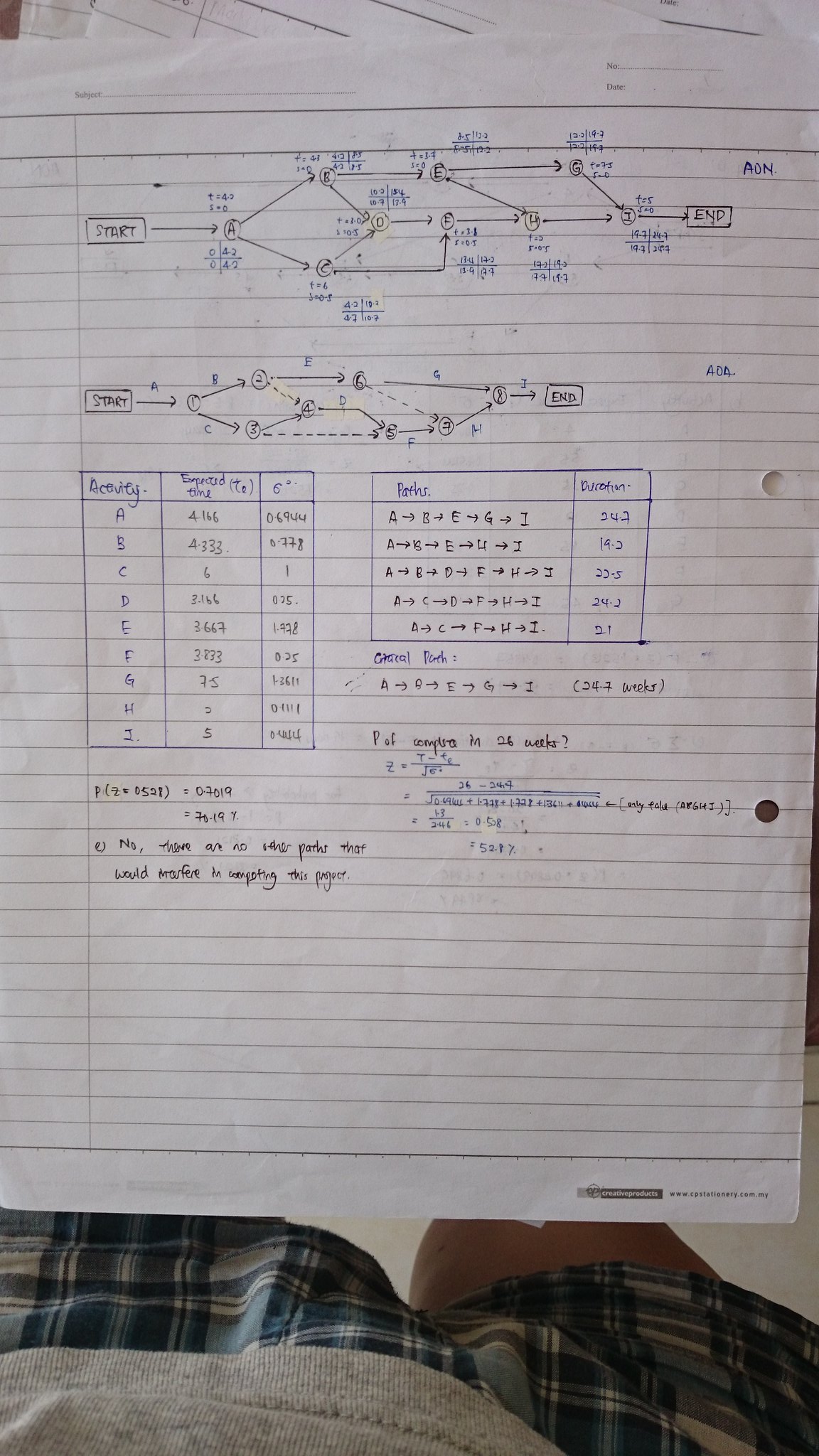This is a photograph of a page from an exercise book, captured by someone standing next to it. The person appears in the frame, showing their tartan pattern shorts and the bottom edge of their gray t-shirt. The page itself is lined and has two diagrams with letters inside circles, connected by directional black arrows. On the left side of the first diagram, there is a box labeled "Start," which connects through arrows all the way to the letter "J." From the circle labeled "J," a black line points to the word "N" inside another black-outlined rectangle. Beside the diagrams, there is a blue 2x2 grid with some numbers.

Below the diagrams, a table is visible with three columns. The first column lists letters from "A" to "J," and the subsequent columns contain two corresponding values for each letter. Further down the page, there are additional mathematical workings and algebraic computations written in both blue and black ink. The exercise book has lines and two holes punched on the right edge, indicating it can be placed in a binder.